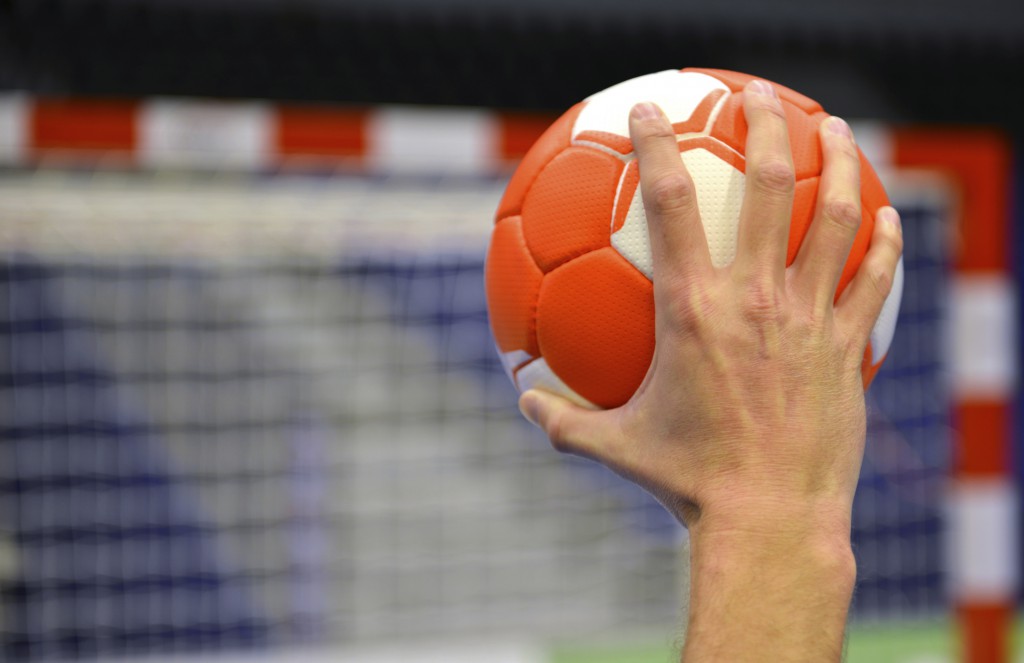In a rectangular image, predominantly wide, a large Caucasian man's hand is prominently featured on the right, holding an orange and white soccer ball with his fingers and thumb spread out. His fingers reveal the pressure applied, as indicated by the light coloration of his knuckles. The background reveals the setting as a soccer field, with the goal net outlined in alternating bands of red and white posts extending vertically near the right-hand side of the image and then turning horizontally across the top. The net itself is tinged blue, with scattered blurry white areas partially obscuring it. Above the net, the darkness suggests a nighttime scene, contrasting with patches of green grass at the lower right and the presence of stadium seating visible as blue and gray sections behind the net, likely indicating blue seats and gray stairs common in stadiums.